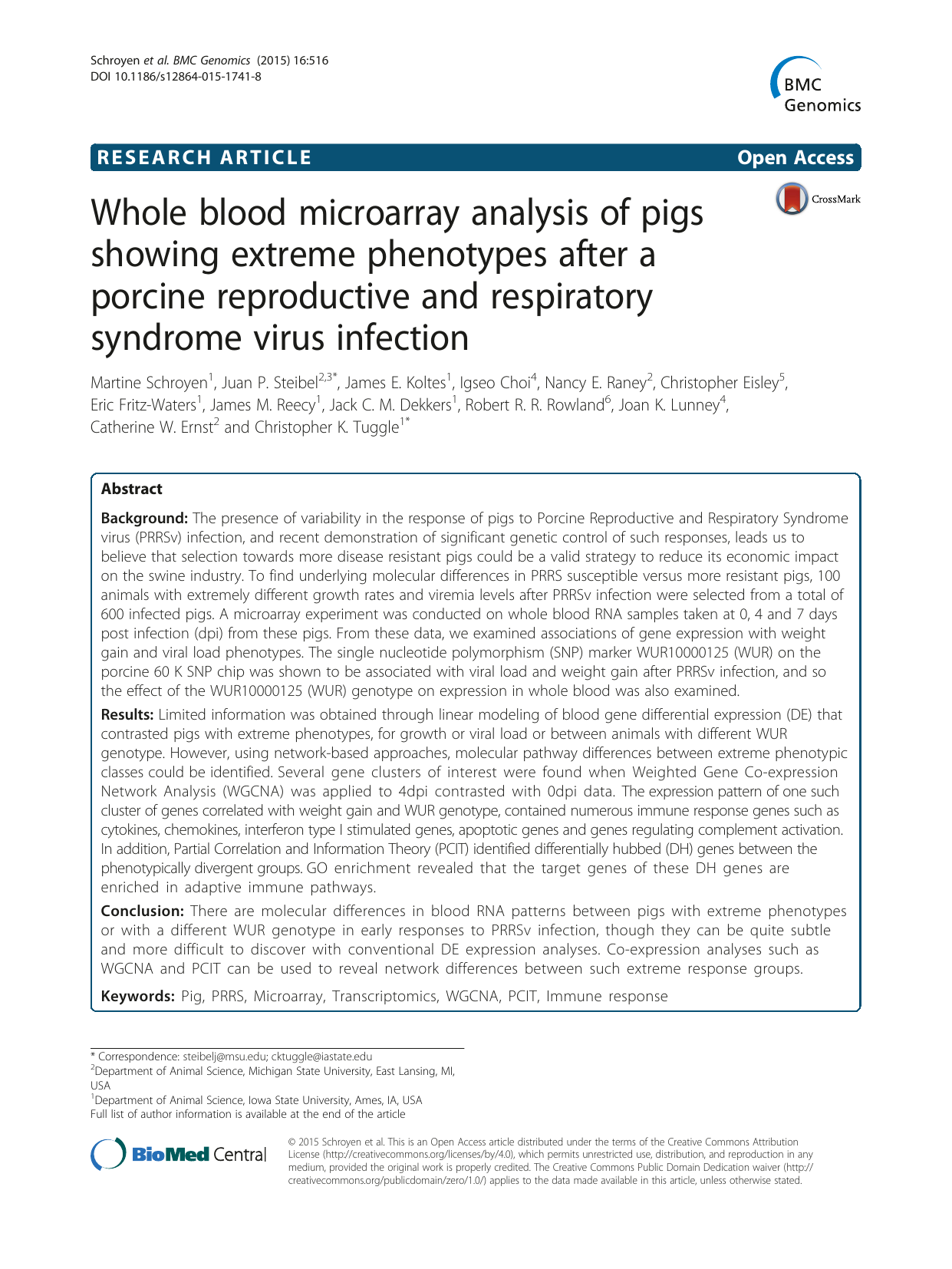This image features a page from an article published in BMC Genomics. At the top right of the page, "BMC Genomics" is prominently displayed. Below that, to the left, the words "RESEARCH ARTICLE" are written in white capital letters against a blue background. On the same blue line, to the far right, the words "Open Access" appear, with only the 'O' and 'A' capitalized, also in white.

The title of the article, situated below this header, reads: "Whole blood microarray analysis of pigs showing extreme phenotypes after Porcine Reproductive and Respiratory Syndrome virus infection." The names of the authors follow the title, listed across three lines in faint gray text.

Further down, there is a boxed section with a white background and a blue border. Within this box, the word "Abstract" is bolded. Below a skipped line, the word "Background" begins the section introducing the research.